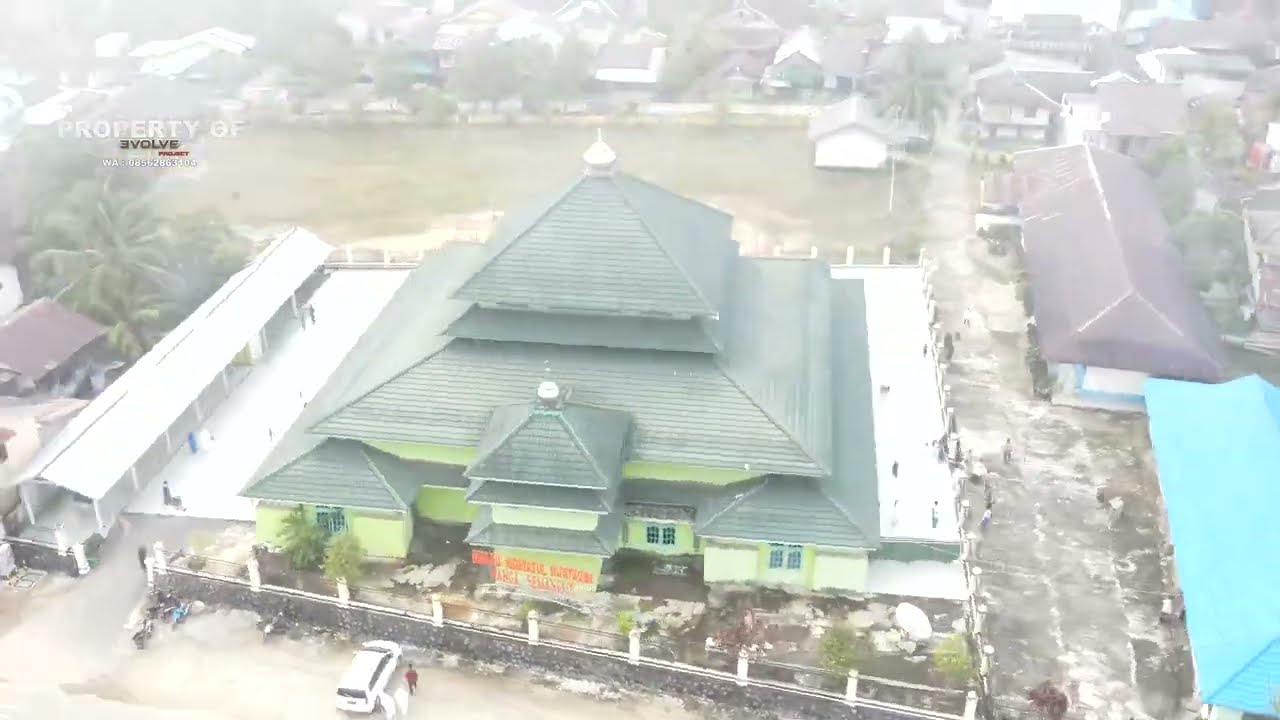An aerial image showcases the expansive Masjid al-Ahsan Mosque in Pemangkat, Indonesia, prominently located amidst a variety of smaller buildings. The mosque features a tiered architectural design with multiple levels of greenish-gray roofs culminating in layered, pyramid-like structures. At the very top, a white spire steeple punctuates the intricate roofline. The minty green sides of the mosque are accented by a red banner with indistinct orange writing.

Encircling the mosque is a robust stone wall with a gated entrance, suggesting a measure of security. Within the premises, the landscaping is meticulously arranged with rocks, small trees, and tropical palm trees that contribute to a serene ambiance. Just outside the fence lies a cement road and parking area where a white vehicle is stationed, and three individuals are engaged, two in white attire and one in red.

The surrounding area is characterized by a mix of single-family homes and other structures with varying roof colors, including brown and bright blue. In the backdrop, a grassy or muddy field is visible, likely used for athletic or celebratory events. This area transitions into a more residential neighborhood. On the left side of the image, an elongated open-air structure with a metal roof is noticeable, adding to the eclectic architectural mix.

The overall setting conveys a warm climate, as evidenced by the sparse yet significant presence of palm trees and the attire of the inhabitants. A subtle watermark in the upper left corner of the image reads "Property of Evolve Project," with contact details displayed beneath it.